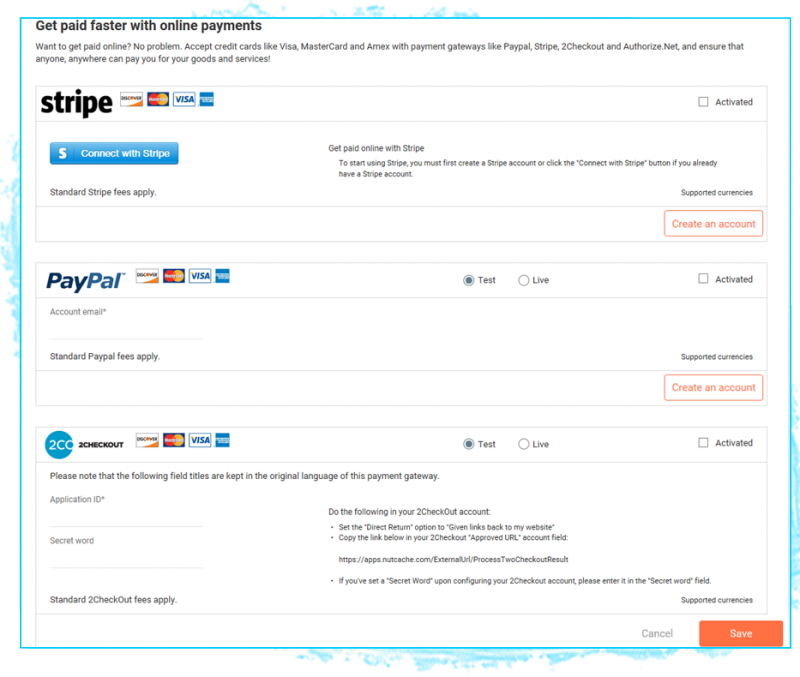The image showcases a section of a website dedicated to online payment services, prominently featuring Stripe and PayPal as payment gateways.

On the left side, the Stripe section is displayed. It conveys the benefits of using Stripe for faster online payments, highlighting its compatibility with major credit cards such as Visa, MasterCard, American Express, and Discover. The section emphasizes that Stripe enables anyone from anywhere to pay you for goods and services. Positioned below the main text is a blue button labeled "Connect with Stripe" in white font, inviting users to link their Stripe account. Additional information clarifies that standard Stripe fees apply. Beside this, a checkbox labeled "Advanced" remains unchecked, and a support link for current supported currencies is provided. A white button with a red border and red text labeled "Create an Account" is also available for new users.

To the right, the PayPal section mirrors similar functionalities. It displays icons for Visa, MasterCard, American Express, and Discover alongside text stating “Account Email” to identify the required information for PayPal transactions. This section also notes that standard PayPal fees apply.

Overall, the image effectively communicates the ease and practicality of accepting online payments through these popular gateways.